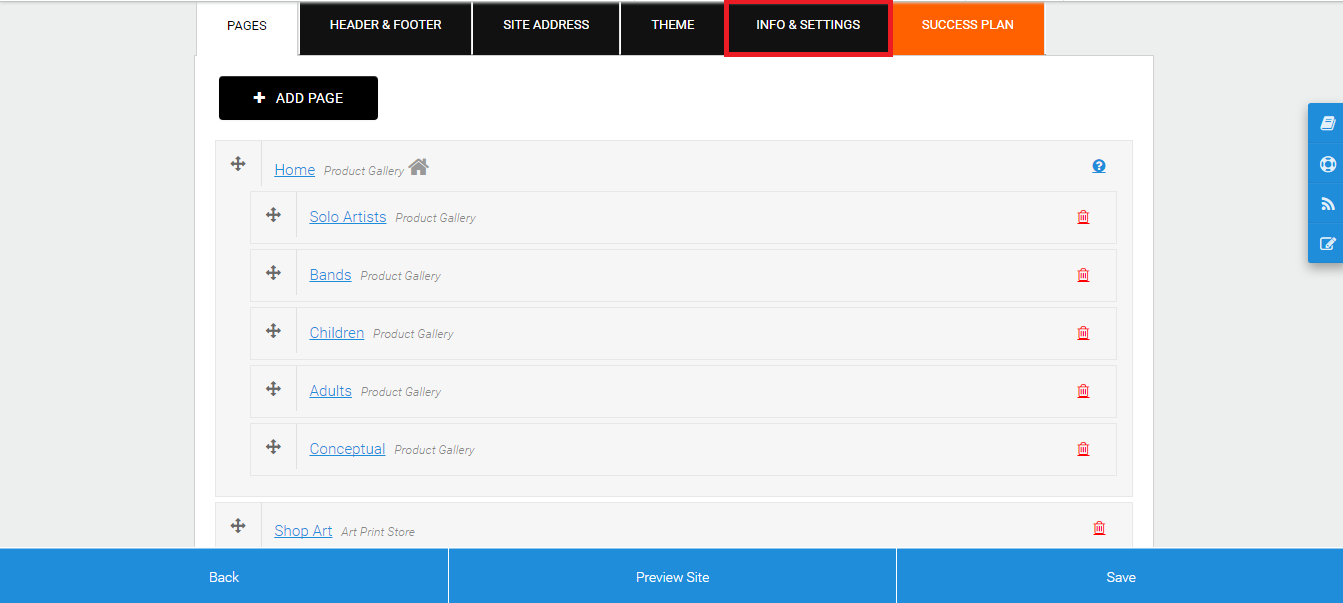The screenshot depicts an interface, possibly from a web development tool or a search engine tailored for website creation, against a white background. The bottom portion of the screen features three prominent blue buttons sequentially labeled: "Back," "Preview Site," and "Save."

On the right-hand side of the window, a small blue banner with four vertically aligned white logos is attached. The main area of the screen displays several selectable options. At the top, there are six tabs: "Pages," "Header and Footer," "Site Address," "Theme," "Info and Settings," and "Success Plan." The "Pages" tab is currently active and in view.

Dominating the top section of the active tab, a large black button with white text reads "Add Page." Below this button, seven categories that users can add are listed vertically: "Home," "Solo Artists," "Bands," "Children," "Adults," "Conceptual," and "Shop Art." Each category row is accompanied by a column of colored icons on the right. The "Home" category features a blue circle with a white question mark, denoting additional information or help. The remaining categories each have a small red icon at the end of their respective rows.

The fifth tab, "Info and Settings," is distinctly highlighted in red, suggesting it may be the most recent or an important area requiring attention.